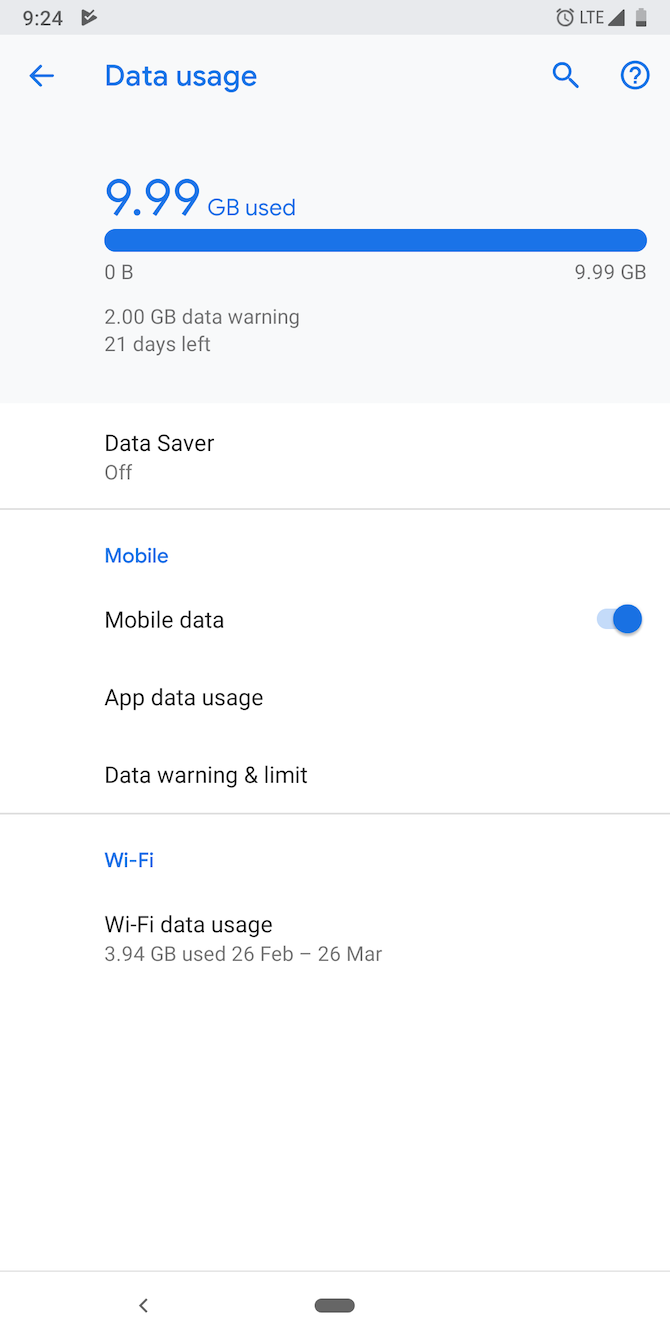The image shows a screenshot of a smartphone’s data usage page. In the top right corner, there are icons indicating the Wi-Fi signal, LTE connectivity, battery level, and other typical smartphone indicators, confirming it is a phone. The main background of the settings page is white, with text primarily in light blue and black for contrast. The user is in the "Data Usage" section of the settings, which displays that they have utilized the full 10 gigabytes of their data plan with only 2 gigabytes remaining before hitting their data cap. The screenshot also notes that there are 21 days left in the billing cycle. At the bottom of the page, there is information about Wi-Fi data usage, indicating that when connected to Wi-Fi, the data usage from the phone service is not counted, affording the user a form of unlimited data while on Wi-Fi.